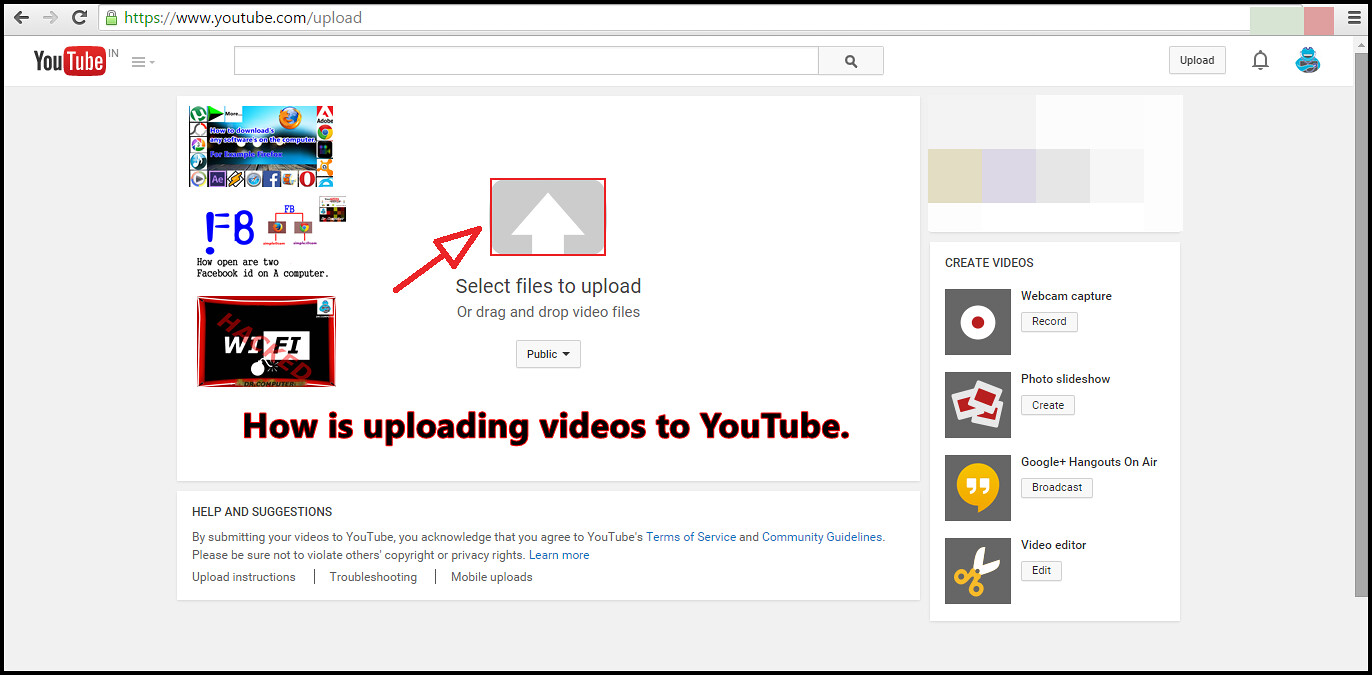The image depicts a computer screen showcasing the YouTube upload page at the URL "https://www.youtube.com/upload." At the top, a long, narrow search bar is visible with a magnifying glass icon on its right side. Adjacent to the search bar is an "Upload" button, followed by a bell-shaped notification icon and another blue icon, which is indistinguishable.

On the left side of the screen, there is a small rectangular illustration containing a photographic image at its center, surrounded by various icons including Facebook and Chrome. Due to their small size, the other icons are not clearly identifiable. Below this illustration, text appears to mention Facebook on one computer, though the exact wording is unclear. 

Further down the screen, a prominent red-bordered black box is displayed with the word "Wi-Fi" and a red crosswise text that might say "Hacked," though it is difficult to discern. A red arrow points upwards towards a red-bordered rectangle containing a white upward-pointing arrow. This section instructs users to "Select files to upload or drag and drop video files." 

Below this instruction, there is a dropdown menu, possibly labeled "public" or something similar, suggesting visibility options for the uploaded video. Text present indicates "How is uploading videos to YouTube," potentially referring to either a guide or a user's activity.

On the right side, a menu related to video creation is visible. The options listed include: 

- Create Videos
- Welcome
- Capture
- Record
- Photo Slideshow
- Create
- Google Hangout (something or other)
- Video Editor

Each option is accompanied by illustrative icons to their left, with the Video Editor option featuring an edit button and a pair of scissors icon.